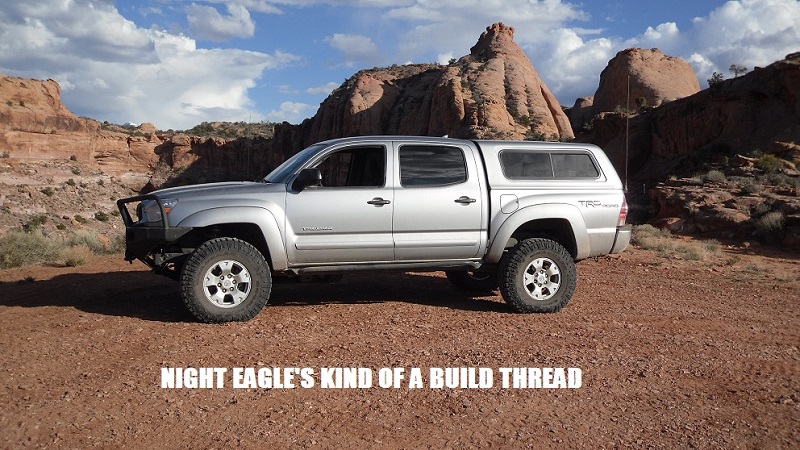In this photograph, styled as an advertisement, a silver extended cab SUV with matching silver hubcaps and black tires is prominently displayed, parked on a surface of dirt and sparse brown soil. The vehicle is oriented with its front to the left and rear to the right, occupying a central position in the image. Behind the SUV, a series of rugged stone cliffs rise, with the tallest, centrally placed cliff distinctly shaped like a triangle. The backdrop features a mix of blue sky and scattered white fair-weather clouds, creating a picturesque outdoor setting.

Below the vehicle, text in bold white capital letters reads, "KNIGHT EAGLES," followed by a tagline, "kind of a build tread," suggesting ruggedness and durability. Subtle patches of grass add a touch of greenery to the otherwise earth-toned foreground, enhancing the natural and adventurous ambiance.